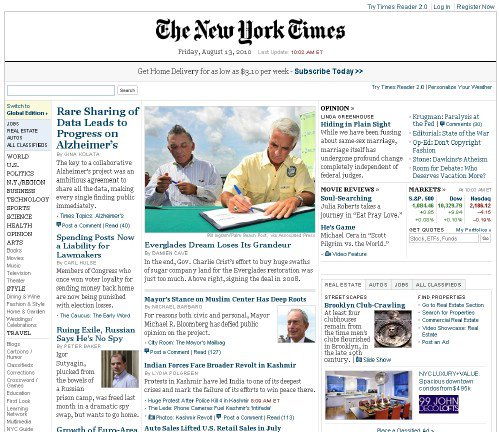**Screenshot of The New York Times Website - Friday, August 13, 2010**

This screenshot captures a segment of The New York Times website dated Friday, August 13, 2010. The interface has a slightly vintage appearance, reflecting design aesthetics from over a decade ago. 

Prominent in the center is the main headline: "Everglades Dream Loses Its Grandeur." Above this primary story, a subscription offer encourages readers to "Get home delivery for as low as $3.10 per week," with a hyperlink to subscribe.

To the top left of the main story, there's a headline reading "Rare Sharing of Data Leads to Progress on Alzheimer's." Directly below this, another article titled "Spending Posts Now a Liability for Lawmakers" is featured. Following in succession is the headline "Ruling in Exile, Russian Says He's No Spy."

Beneath the central Everglades story, another article titled "Mayor's Stance on Muslim Center Has Deep Roots" is highlighted. There is also an image of Mike Bloomberg, reflecting the political landscape and notable personalities of the period.

This snapshot provides a rich tapestry of news topics from 2010, illustrating a moment in time through its careful assembly of headlines and visuals.